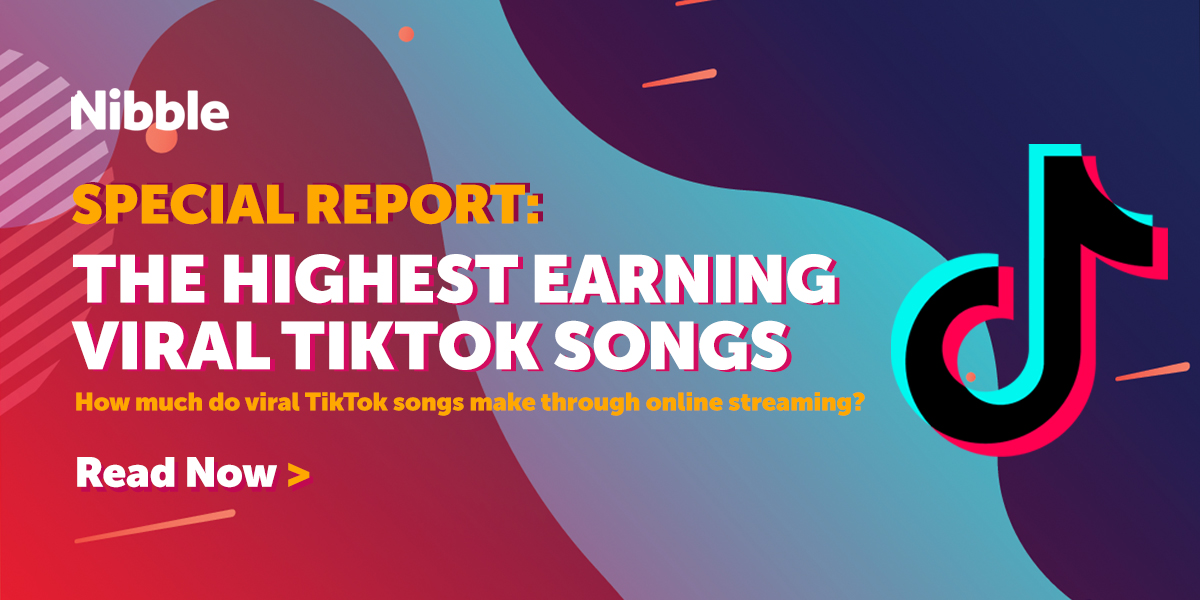Caption: 

"Nibble Special Report: The Highest-Earning Viral TikTok Songs - Explore How Viral TikTok Songs Generate Income Through Online Streaming"

Description: 

The image features a TikTok symbol positioned to the left side, intricately detailed in black with complementary blue and red highlights—blue on the left and red on the right. Behind the symbol, a swirling blue blob of color forms the dynamic background, which transitions into black in the top right and bottom left corners. Additionally, the bottom left corner radiates a subtle red hue that glows and enhances the visual complexity. The text, presented in a striking mixture of yellow and white, draws attention to the report's key insights.